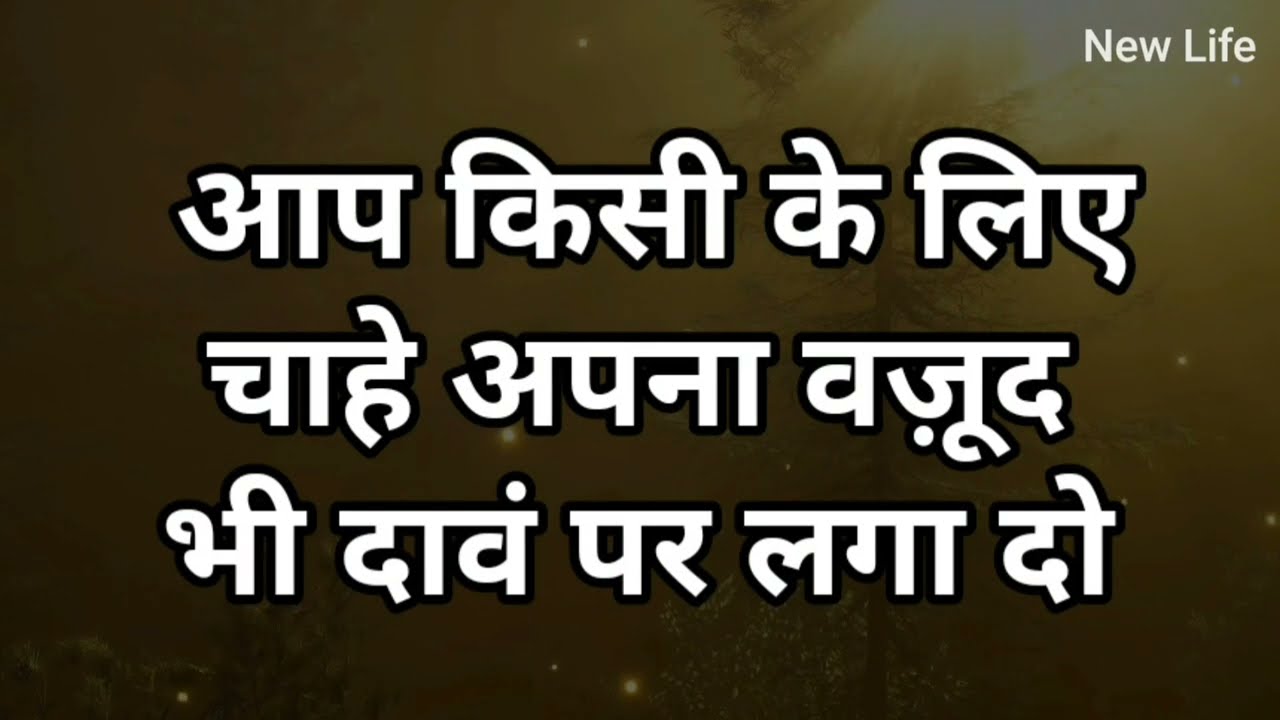The image presents a hazy, dark scene with a muddy brown hue permeating the background, suggesting a setting perhaps clouded by wildfire smoke or other environmental obscurities. The upper right corner of the image shows sunlight piercing through the murkiness, partially illuminating a tree that stands against the otherwise dark and brown backdrop. Across the image, in three rows, bold Arabic text in white font bordered by black stands prominent. The first row consists of four words, the second row has three, and the third row displays five words. These characters potentially depict a religious quote or an important statement, though their exact meaning is unclear. Above this foreign text, in the upper right corner, the English words "New Life" are clearly visible in white font, subtly suggesting themes of renewal or hope amidst the obscured scene.